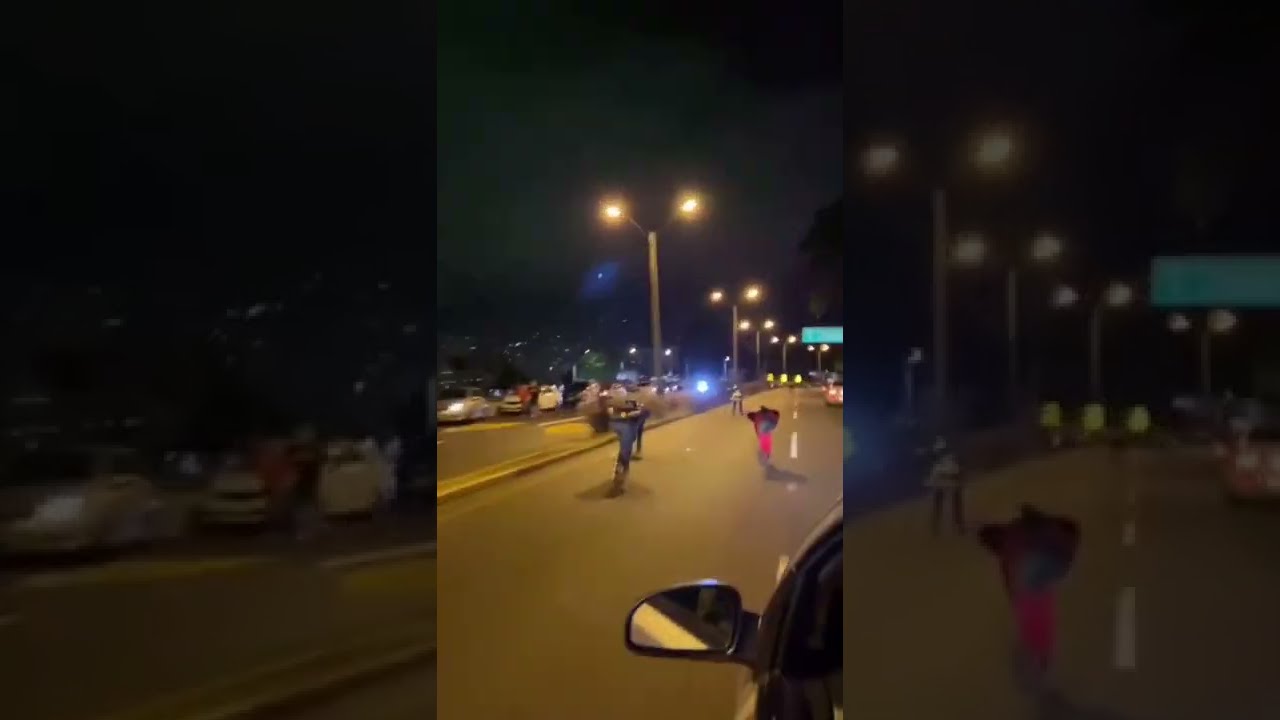This nighttime photo, likely taken from a vehicle or motorcycle in motion, captures a blurry view of a highway divided into three segments. The left and right sides are noticeably out of focus, perhaps due to motion or enlargement, while the middle section is clearer. The lower right corner reveals part of a vehicle, specifically the left-side mirror, suggesting the photographer's vantage point. The scene ahead features a road with two lanes divided by a dotted line. In the middle of the street stands a person wearing a pink outfit, their purpose unclear. Nearby, someone appears to be performing a wheelie on a motorcycle. Further down the highway, a row of streetlights illuminates the path, punctuated by various vehicles. On the right side, a car with headlights on is stopping, while another car approaches from the distance. The left side reveals additional blurry cars, indicating oncoming traffic. The image, despite its blur, vividly depicts a dynamic night-time highway scene filled with vehicles and scattered individuals.